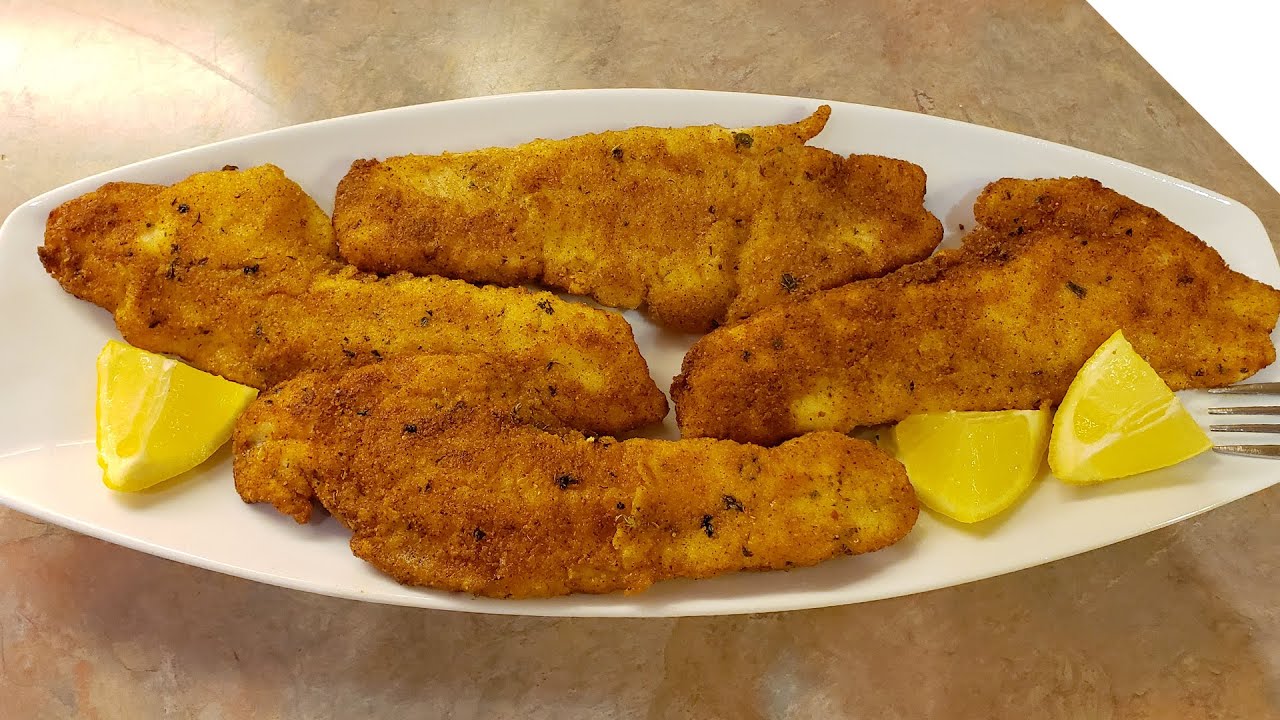This is a close-up photograph featuring four breaded and browned fish fillets arranged on an oval, white ceramic plate. The fillets, shaped like inverted triangles, appear seasoned with visible green herbs, possibly parsley. Surrounding the fish are three lemon wedges, adding a burst of color. The plate is positioned on a brown tabletop, with the edge of the table slightly visible. A silver-colored fork is partially seen at the lower right edge of the image. The background remains clear and white, drawing full attention to the neatly presented dish.